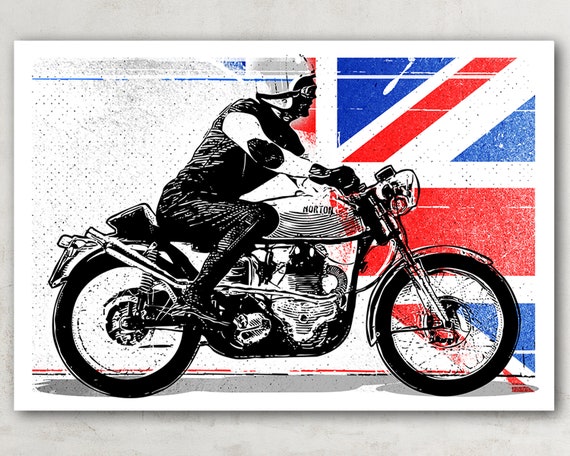The image portrays a detailed illustration that appears to be either a computer-generated print or a hand-drawn sketch, likely intended for sale and suitable for hanging on a wall. The entire composition is set against a light gray background with a crisp white border. Dominating the scene is a black-and-white sketch of a man on a motorcycle, facing right. The rider is outfitted in a suit with black gloves, a white helmet, and black goggles, exuding a classic, monochromatic look. The motorcycle itself bears the name "Morton" on its side. In the background, the right side displays a fragmented representation of the British flag, rendered in dots of red, blue, and black, adding a splash of color behind the rider, while the left side of the background fades to black and gray dots on a white expanse. This sophisticated artwork does not feature an artist's signature, making the name on the motorcycle the only identifying mark.